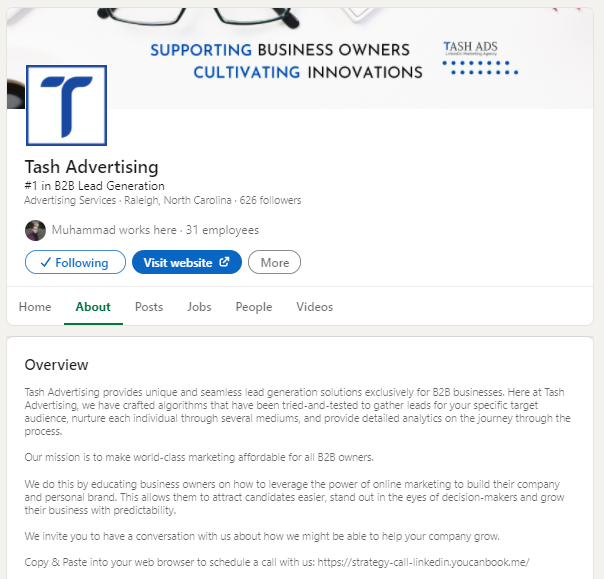This image is a screen capture of a website for Tash Advertising. The design follows a clean layout with a primarily white background complemented by black text and light gray banners framing the sides and top of the page. 

At the top, there is a prominent banner featuring a photograph of a light gray desktop adorned with a pair of black eyeglasses. Beside the image is a tagline in blue and black text that reads, "Supporting Business Owners, Cultivating Innovations." Situated to the right of this is the Tash Advertising logo, followed by two rows of small dark blue dots that add a touch of elegance and structure to the layout.

Below this banner, on the left side, there is a square icon featuring a stylized blue 'T,' which serves as the logo for Tash Advertising. To the right of this icon, black text reads, "Tash Advertising," followed by the tagline "Number one in B2B lead generation, Advertising Services," and the location details, "Raleigh, North Carolina." It also mentions that the company has "626 followers."

Additionally, there is a brief mention that an individual named Muhammad works here, and the company has 31 employees. Below this information, there are action buttons labeled "Following," "Visit Website," and "More," ensuring easy navigation and user interaction.

Further down the page, there is a horizontal navigation bar with tabs for "Home," "About," "Posts," "Jobs," "People," and "Videos." The "About" tab is currently highlighted in green, indicating the user is viewing this section. The "About" section displayed at the bottom portion of the screen includes a heading, "Overview," followed by a detailed write-up about the company's mission, services, and core values.